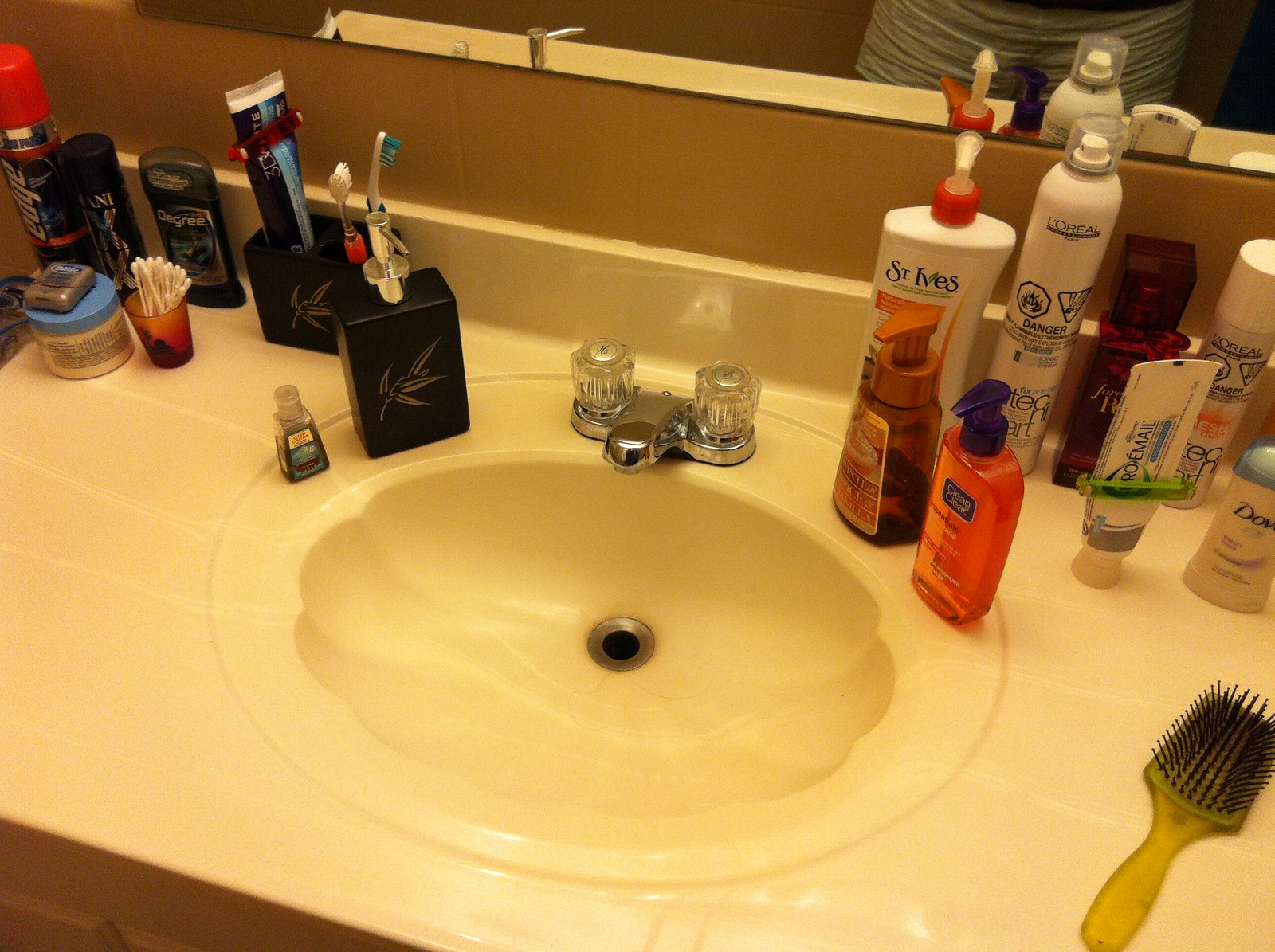This close-up photograph captures a bathroom sink and counter adorned with personal toiletries, reflecting a lived-in, everyday setting. The upper part of the image includes a partial view of a mirror and shows the lower portion of a person wearing white shorts, likely the photographer. The focal point is an oval-shaped sink set into a somewhat dated tan laminate countertop with an off-white hue. Darker tan tiles form a backsplash between the sink and the mirror, adding texture to the background.

On the left side of the sink, an array of men’s grooming items is neatly arranged: a black square soap dispenser, a black container holding toothbrushes and toothpaste, Degree men’s deodorant, a small cup of Q-tips, Glide dental floss, Edge shaving cream with a red cap, and a few other toiletries. 

The right side of the sink showcases women’s products: an orange face wash, possibly an additional soap, St. Ives body lotion, Dove women’s deodorant, Pro-Expert toothpaste, L'Oreal hairspray, a red bottle of an unidentified product, and a yellow-green hairbrush with a square head and black bristles positioned in the lower right corner. The detailed assortment of items gives a comprehensive view of the daily care routines of the occupants.